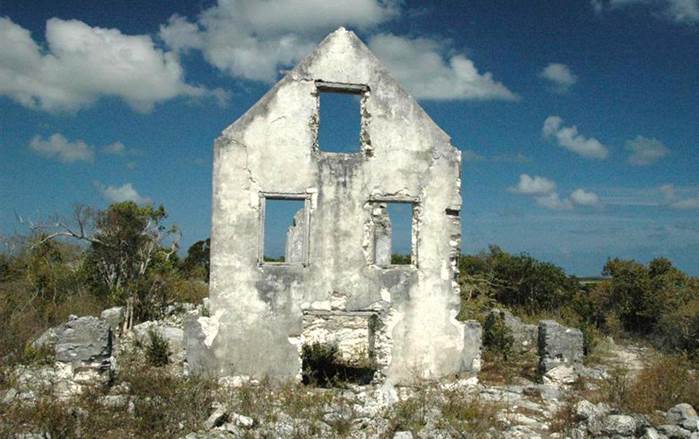The image shows the ruins of an old, deteriorated building, likely a home, standing alone under a clear blue sky with slight cloud coverage. The structure's front face is the only part still intact, displaying heavy degradation with numerous cracks and broken corners. This facade features a triangular arrangement of three windows: one at the top center, and two below it, with an entrance way at the bottom. Surrounding the ruins are rocks and rubble, interspersed with weeds and small green trees. The area is dotted with small bushes, lending a slightly tropical atmosphere to the scene.